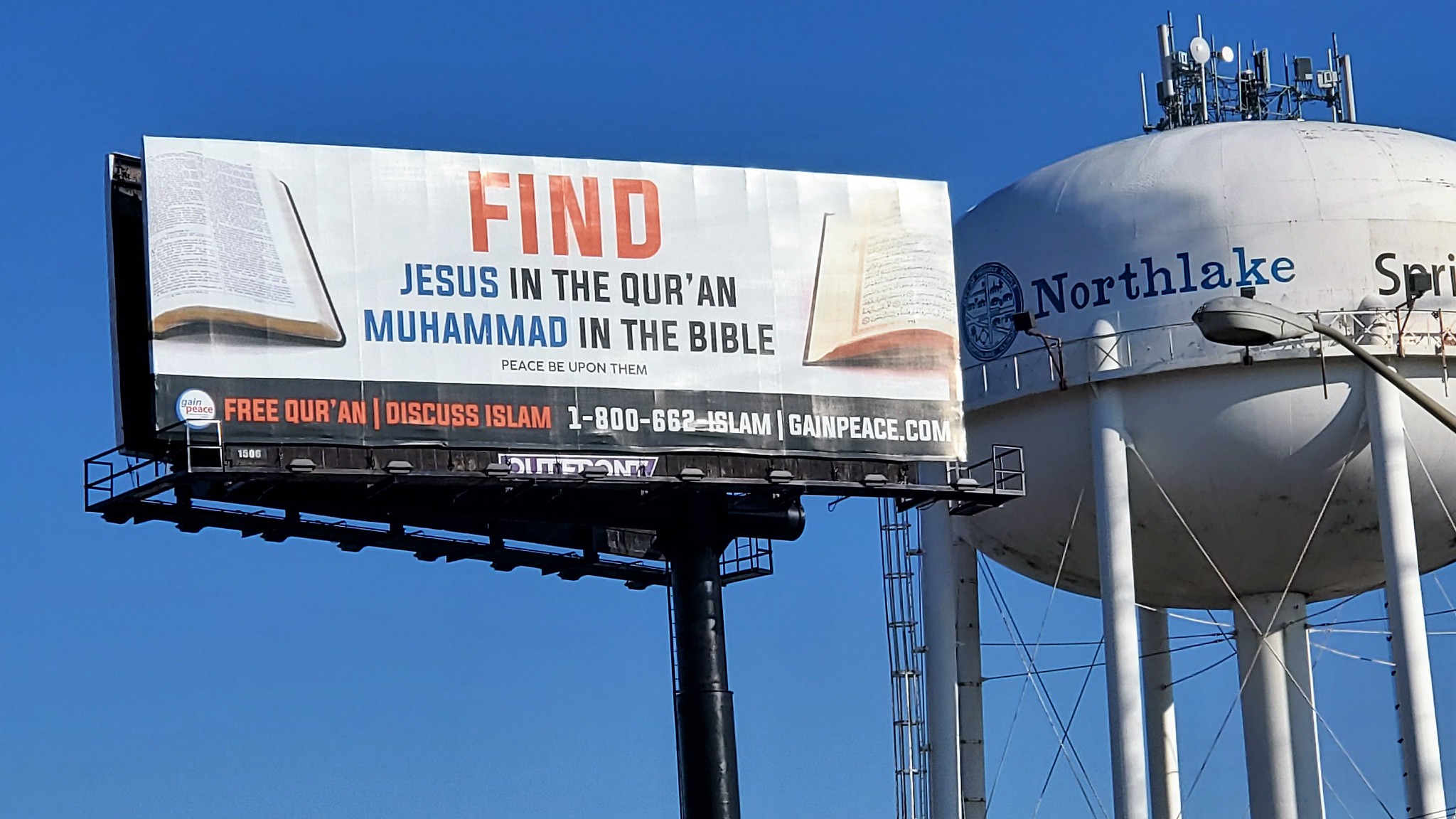The image depicts a large, rectangular billboard set against a clear, bright blue sky. The billboard is primarily white with a prominent message that reads in various colors: "FIND Jesus in the Quran, Muhammad in the Bible, peace be upon them." Flanking this text are open images of a Bible and a Quran. Below the central message, there is a black strip with red and white text promoting a free Quran with the contact details: "FREE QURAN, DISCUSS ISLAM, 1-800-662-ISLAM, gainpeace.com." To the right of the billboard stands a tall, white water tower labeled "North Lake" in blue text, with additional labeling likely part of a seal, and a ladder is visible ascending the structure. The tower is encircled by several wires and lights. The overall scene is devoid of clouds, showcasing a clear and unobstructed sky.